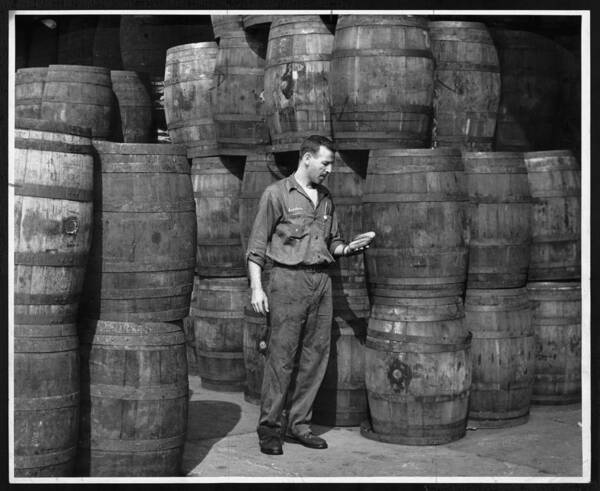In this detailed black and white close-up photograph, a Caucasian male factory worker stands at the center of a room filled with aged wooden barrels. Dressed in a leather denim jacket, matching leather denim pants, and black sole boots fastened with a black belt, he epitomizes a meticulous worker. His clean-cut hairstyle adds to his sharp, focused demeanor as he inspects an indeterminate object in his left hand. The worker's shirt is buttoned up, leaving only the first two buttons undone. Surrounding him are numerous barrels, some stacked up to four high, varying in light and dark shades of gray, indicating their different colors in real life. The barrels, appearing several decades old, suggest they possibly hold fermented liquids, such as alcohol, although no labels confirm their contents. The barrels number between 30 to 40 in a room characterized by a hard concrete floor and an obscure black background, emphasizing the age and setting of this industrial scene.